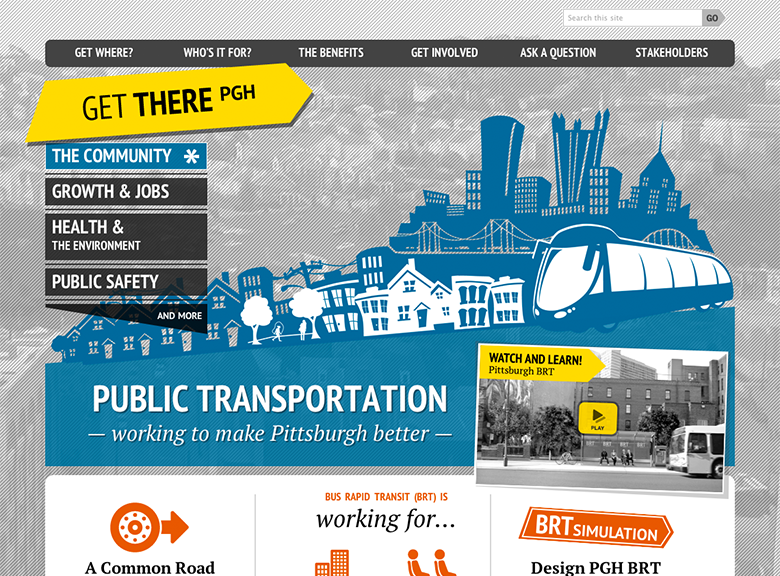The webpage of the website prominently features several navigational tabs at the top, including "Get Where," "Who's it For," "The Benefits," "Get Involved," "Ask a Question," and "Stakeholders." Above these tabs is a search box accompanied by a "Go" button. Immediately beneath this navigation bar, a striking yellow banner displays the label "Get There PGH" with secondary tabs categorizing content for "Community," "Growth and Jobs," "Health and the Environment," "Public Safety," and more.

An animated graphic in blue and white provides a stylized representation of a cityscape. This graphic prominently features both a city skyline and a residential area, alongside a public transportation bus, underscored by the text "Public Transportation: Working to Make Pittsburgh Better."

To the right of the image is an embedded video titled "Watch and Learn! Pittsburgh BRT," with a large play button situated in the middle of the preview screen. The video appears to depict a different era in black and white, showing a classic city bus in front. 

Beneath the video, an icon is displayed followed by the text "bus rapid transit BRT is working for..." (with an ellipsis indicating continuation). Below this text are graphics representing various elements such as buildings and an icon of two people seated as if on public transportation.

The page concludes with a banner dedicated to "BRT Simulation," highlighting the design of the "PGH BRT" initiative.